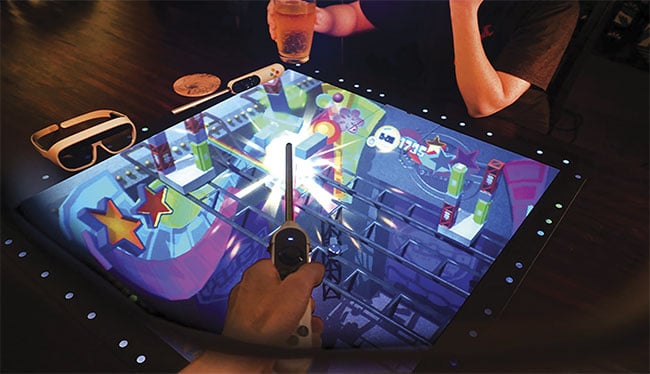The digital image captures two people engrossed in a tabletop bar video game, which features a vibrant display directly on the tabletop surface. One player, identifiable by his brown or black t-shirt, is partially visible with his torso and arms shown. He holds a beverage, likely a soda or beer, in his right hand. Resting in front of him are a pair of possibly polarized goggles, hinting at a 3D experience, and a wand-like remote control, which he currently isn't holding. The game table itself is dark, contrasting with the bright, colorful, cartoonish graphics that dominate the screen. The second player, whose white hand is seen near the bottom of the image, grips a similar wand-like control, seemingly interacting with the game's intense central light burst. This light explosion is encircled by red and orange stars and purplish-pink ribbons of color, creating a dramatic visual effect. The game itself features a triangle-shaped interface with a score display reading "1735." The detailed surroundings on the table emphasize additional elements such as another stick control and the gold virtual glasses, all set against the dark table surface, enhancing the immersive gaming atmosphere.